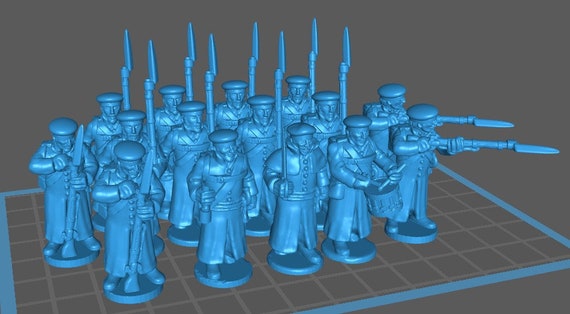This image is a 3D-rendered, digitally created scene with a charcoal gray background. The layout is landscape, with a blue square at the bottom featuring a grid patterned with tan checkerboard lines. On this grid stand numerous blue figurines resembling toy soldiers, detailed much like plastic green army men but more refined. 

These figurines, dressed in European-style military uniforms with flat caps, are posed in various stances: some are holding rifles with bayonets over their shoulders, others appear to be reloading muskets, and a few are actively firing. Resembling World War I or II soldiers, they stand on a tiled board, giving the impression of chess pieces in action. The posing and the setting suggest a concept rendering, potentially for a 3D printing project or similar visual endeavor.